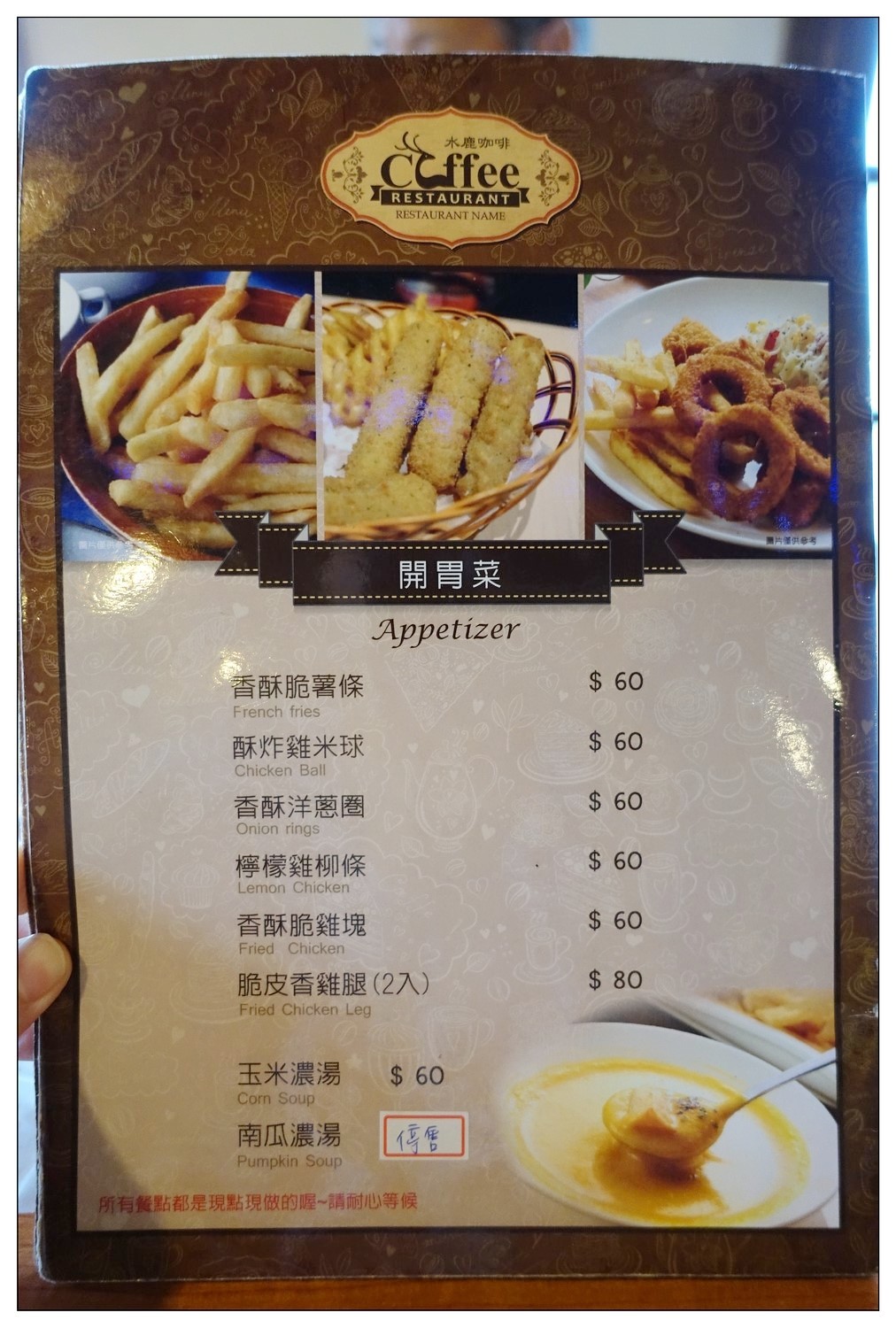This photograph captures a multilingual menu being held by a person, with only their thumb visible at the bottom left corner. The menu is likely from an East Asian country, as indicated by the small text at the top, which could be in Korean, Japanese, or Chinese. The title at the top reads "Coffee Restaurant," with the establishment's name written below in English.

On the menu's top left, there's a section labeled "French Bar." Adjacent to this, in the top middle, is an image of a basket holding a dozen waffle fries, while to the right, one finds onion rings, French fries, and coleslaw, all neatly arranged. 

The central portion of the menu prominently features appetizers, displayed under a black banner with white text. The main text is in the original East Asian language, but English translations are provided underneath in small red text. The listed items include French fries, chicken ball, onion rings, lemon chicken, fried chicken leg, corn soup, and pumpkin soup. Pricing details indicate that most items are priced at 60, except for the fried chicken leg at 80. Notably, the price for pumpkin soup is listed inside a square writing box and is the only item without an English translation.

In the bottom right of the photograph, there is an image of a bowl of soup. The detailed and organized layout of the menu suggests a blend of Americanized food offerings within an East Asian culinary context.